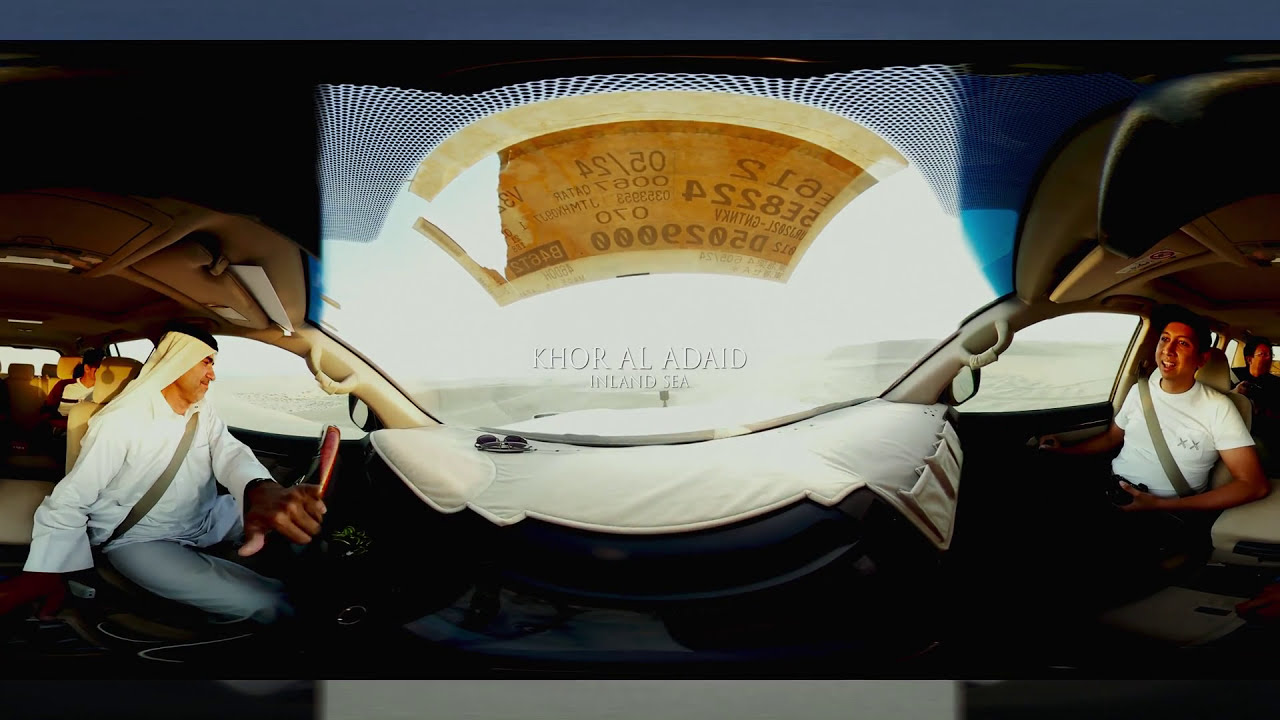The image depicts a scene inside a car, split vertically down the middle, providing a wide-angle view akin to a stitched-together screenshot from a dash cam or action camera. On the left side, the driver, who is dressed in traditional Middle Eastern attire with a white headdress and matching long sleeves, grips a red steering wheel while restrained by a tan or gray seatbelt. Behind him, a passenger in a white outfit with a black stripe is partially visible. On the right side, the front-seat passenger wears a white t-shirt with two Xs on the pocket and dark pants, his arm resting on a tan central console. This person appears to be holding a black object, possibly a camera. Seated behind him is another passenger wearing glasses and dark clothing. 

The dashboard is cluttered with items, including a white cloth with pockets and a pair of sunglasses. The windshield features a yellow sticker filled with various numbers and letters, visible in reverse from inside the car. Prominently displayed above the sticker is the text "Khor al-Adeid Inland Sea" in white letters with a thin black shadow. Outside the car, the environment resembles a white sand desert, suggesting a remote location.